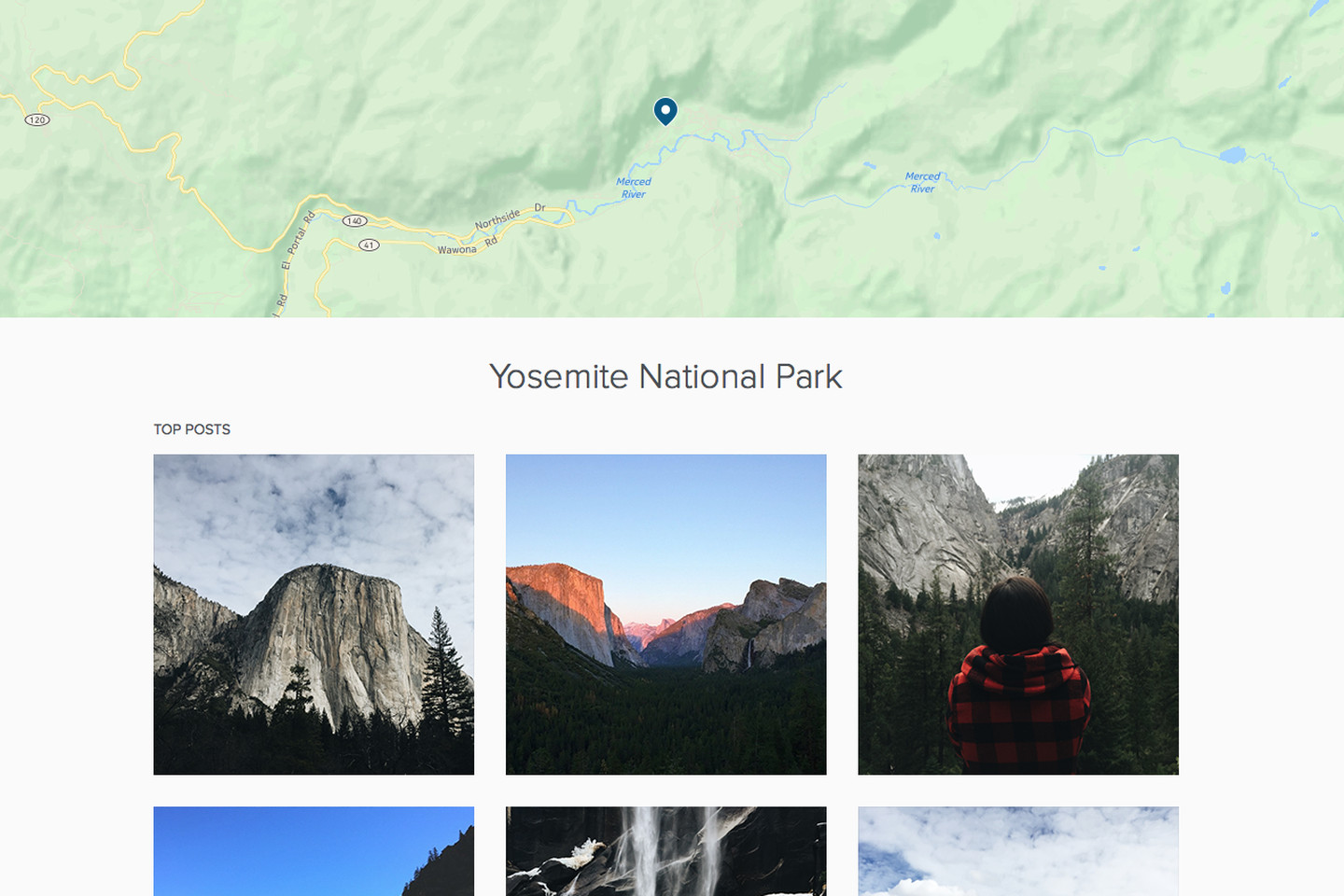A detailed review of Yosemite National Park is visually summarized in this multi-layered image. At the top, a banner displays a simplified and nearly detail-free map pinpointing Yosemite Park’s location. This map, though minimalistic in road details, effectively uses relief shading to suggest the park's varied topography and elevation changes, offering a quasi-3D perspective. Below the map, the text "Yosemite National Park" is unassumingly printed in regular font, notably not bold, which might seem odd for a headline. Beneath this text, the section titled "Top Posts" showcases a collection of notable visitor photographs. The first row features three striking images of Yosemite's iconic stone formations, with the third photo capturing a child gazing up in awe at these natural structures. The lower row hints at additional intriguing images, though they remain partially obscured, inviting viewers to scroll down for a better view.